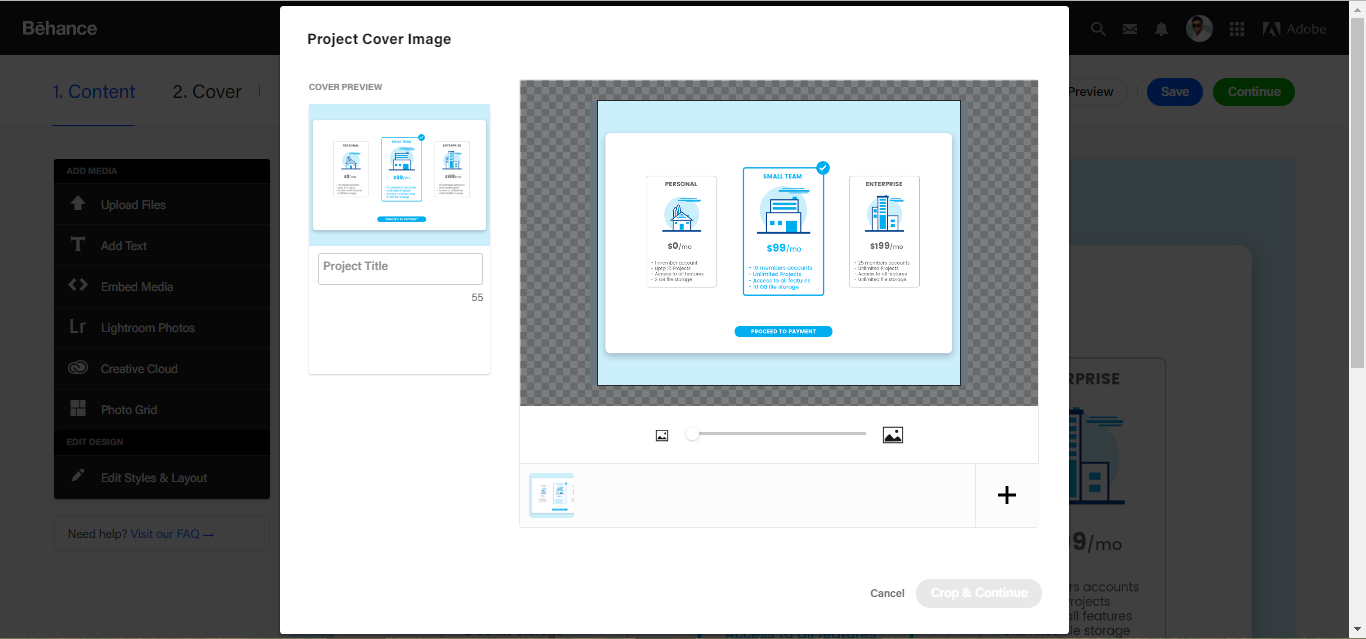The image displays a computer screen, predominantly showcasing the Behance website interface. In the top black toolbar, the word "Behance" is prominently displayed. To the right of the word "Behance," there are several icons: a magnifying glass, a mail message icon, a bell notification icon, and a profile picture of a person wearing sunglasses. Adjacent to these icons are nine dots arranged in a grid pattern.

Below this toolbar, there is a blue highlighted tab labeled "Content" alongside another tab labeled "Cover," although the rest of the tabs going across are obscured. On the far right side of this section, there are three buttons: "Preview" in white, "Save" with a blue background, and "Continue" highlighted in green.

On the left side of the screen, there is a vertical black box containing various options: "Upload File," "Add Text," "Embed Media," "Create Room," "Photos," "Creative Cloud," and "Photo Grid." At the bottom of this box, it instructs users on "Easy stylus and layout" with an additional prompt that says "Need Help? View our FAQ."

Overlaid on this background is a white screen section titled "Project Cover Image," showcasing three different options each with varying prices, though the text size makes the details hard to discern. This section also includes "Cancel," "Copy," and "Continue" buttons at the bottom.